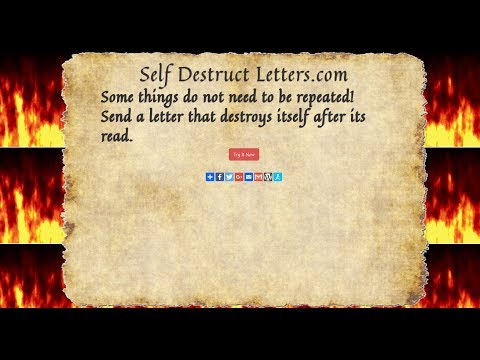This image features a tattered, off-white parchment paper as the central focus, set against a dramatic backdrop of three identical horizontal rows of simulated flames. The flames are bright yellow at the base, transitioning to red as they ascend, creating a vivid contrast against the jet-black background that frames the top and bottom of the image. The parchment paper, with its ripped and uneven edges, takes up the majority of the image and contains text in a classic, black font. At the top of the parchment, the heading reads "selfdestructletters.com" followed by smaller text: "Some things do not need to be repeated. Send a letter that destroys itself after it's read." Below this message, a prominent red button with white text boldly invites the viewer to "Try it now." Beneath the button are icons for various social media platforms like Facebook, Twitter, Google+, and Gmail, allowing easy sharing across different networks.